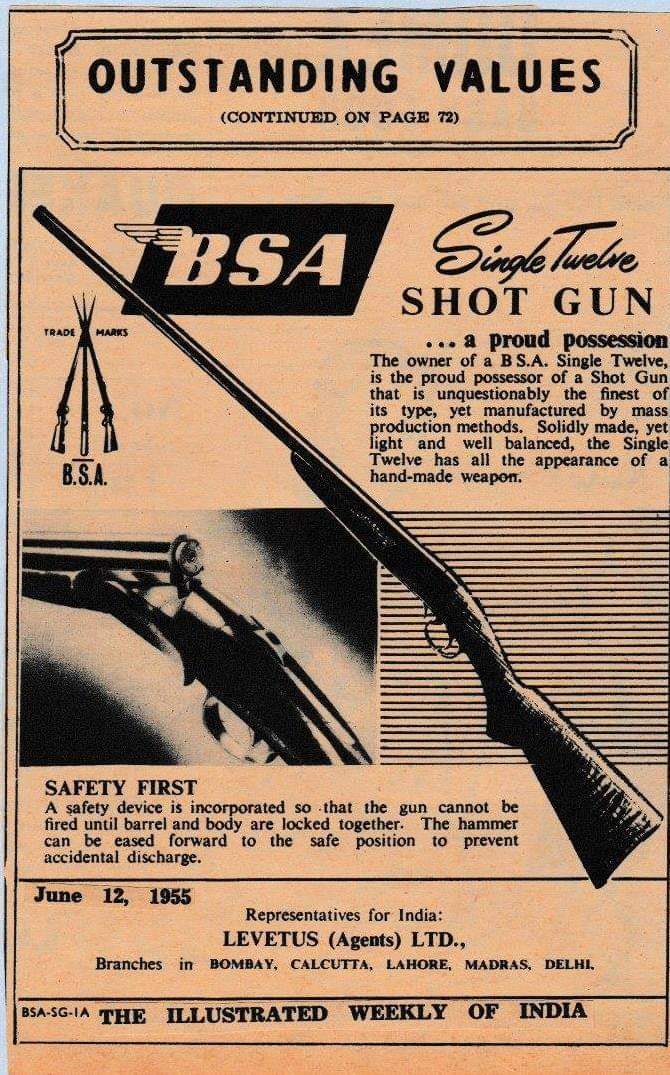This image appears to be a vintage advertisement page from a 1950s magazine, characterized by a salmon-colored background and age-yellowed text. The heading at the top reads "Outstanding Values (continued on page 72)." Central to the ad is an illustrated depiction of a BSA Single 12 shotgun, presented diagonally for an emphasis on its length and craftsmanship, alongside a close-up black and white photograph illustrating the loading area, trigger, and barrel of the gun. The BSA logo, featuring wings on the "B," is prominently displayed alongside a secondary logo depicting three intersecting rifles with the label "BSA Trademarks."

The text describes the shotgun as a "Proud Possession," noting that "the owner of a BSA Single 12 is the proud possessor of a shotgun that is unquestionably the finest of its type, yet manufactured by mass production methods." It emphasizes the shotgun's robust build, balanced weight, and handmade appearance. Safety features are highlighted, explaining that a safety device ensures the gun cannot be fired unless the barrel and body are securely locked together, and that the hammer can be eased forward to prevent accidental discharge. The date "June 12, 1955," is noted, along with details about distribution by Levitas Agents Ltd., with branches in Bombay, Calcutta, Lahore, Madras, and Delhi, presumably connected to "The Illustrated Weekly of India."